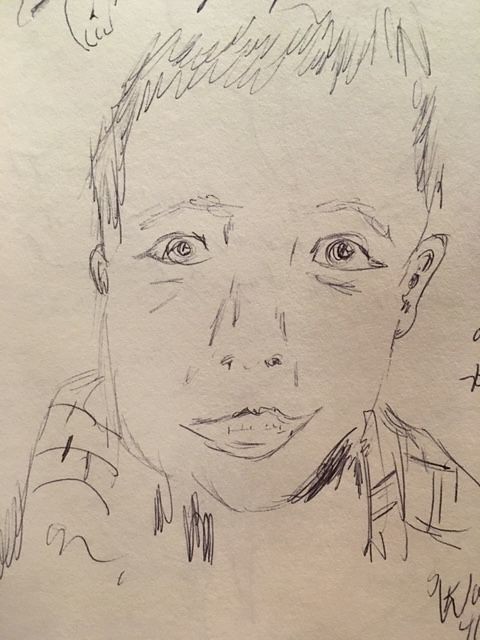In this rectangular pencil sketch, set against a light beige background typical of an artist's sketchbook, we are presented with the face of a young boy. His short hair is meticulously rendered in pencil, featuring distinct bangs that frame his forehead. The boy's eyes are wide and light in color, conveying a sense of innocence and curiosity. His facial features include a small nose and a broad, expressive smile accentuated by his prominent lips. 

The top of what appears to be a plaid short-sleeved shirt is visible, hinting at a casual, youthful attire. While the drawing showcases earnest effort, the execution suggests a beginner's touch, marked by certain imperfections and the raw charm of an amateur artist's hand. A scribble, likely the artist's signature, is located in the lower right-hand corner; although mostly indecipherable, the letter 'W' stands out.

Beneath the boy's neck, a dark shading in pencil adds depth and contrast to the sketch. The right ear is clearly defined, while only the top of the left earlobe is visible. Overall, the sketch captures the essence of a young boy with detailed attention to facial expressions and subtle nuances.